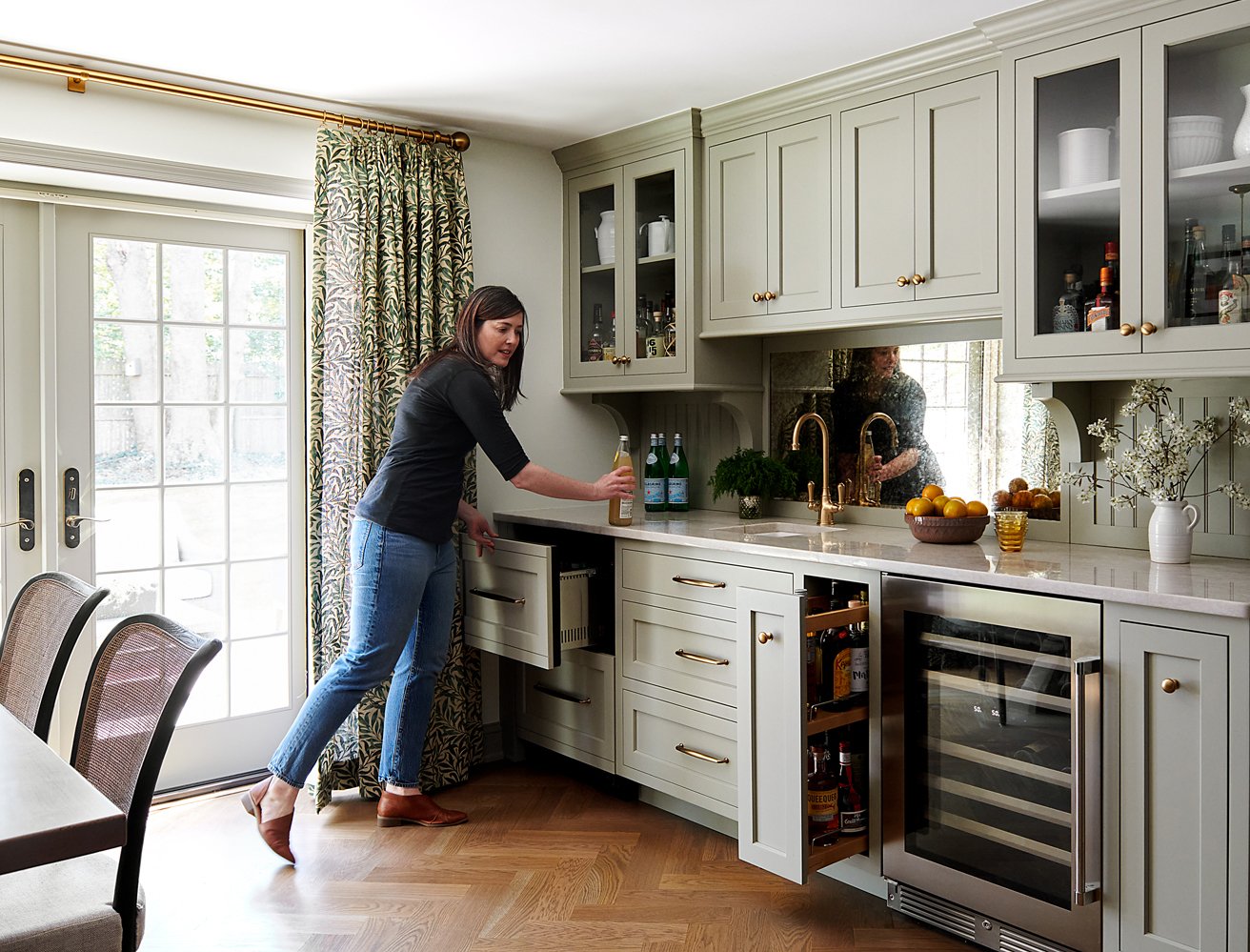In the photograph, a young brunette woman in her 30s, dressed casually in a black shirt, blue jeans, and brown boots, stands in an upscale kitchen and dining area of her home. She is holding a glass bottle of an orange drink by a countertop. The kitchen is adorned with green-gray cabinets, a gold faucet, and matching gold handles on the drawers. There are both upper and lower cabinets, some with clear glass windows displaying various liquor bottles and dishes. Notably, there's a pull-out drawer for wine and more alcohol stored in a bottom drawer. The kitchen also features a bowl of oranges on the counter and three bottles of Pellegrino in the background. The room boasts wooden plank flooring and houses a white table with black and brown chairs. The scene is completed with elegant French doors that have curtains displaying a yellow and green leaf design.